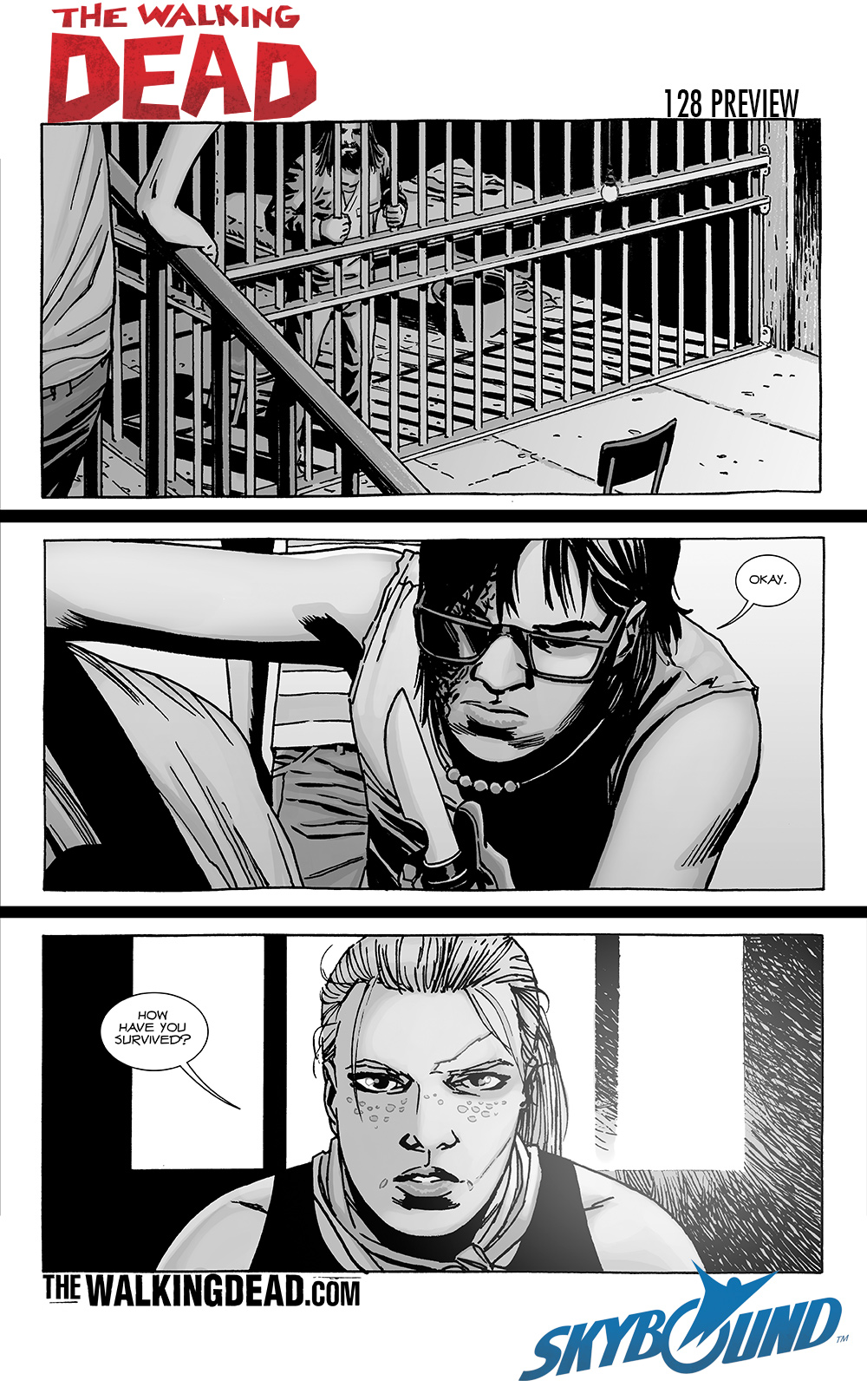This image appears to be a comic book page from The Walking Dead series, specifically a preview of issue 128. The top of the page features "The Walking Dead" in prominent red text, with "128 Preview" in black text on the right. The background is mostly rendered in blacks, grays, blues, and whites.

The page is divided into three panels. The top panel shows a man with long hair and a beard behind bars, gripping them as he looks out. Beside him, a partially cut-off figure stands on a staircase, interacting with the man in the cell. The middle panel features a man crouched down, holding a knife. He has slightly long hair, glasses, a sleeveless shirt, and a necklace, with a word bubble next to him stating, "Okay." The bottom panel depicts a determined-looking woman with blonde hair in a ponytail, standing in front of a window. She has freckles and is wearing a black muscle top. Her word bubble questions, "How have you survived?"

At the very bottom of the image, there are the words "thewalkingdead.com" and "Skybound" in blue text, indicating the publisher and the comic's official website.